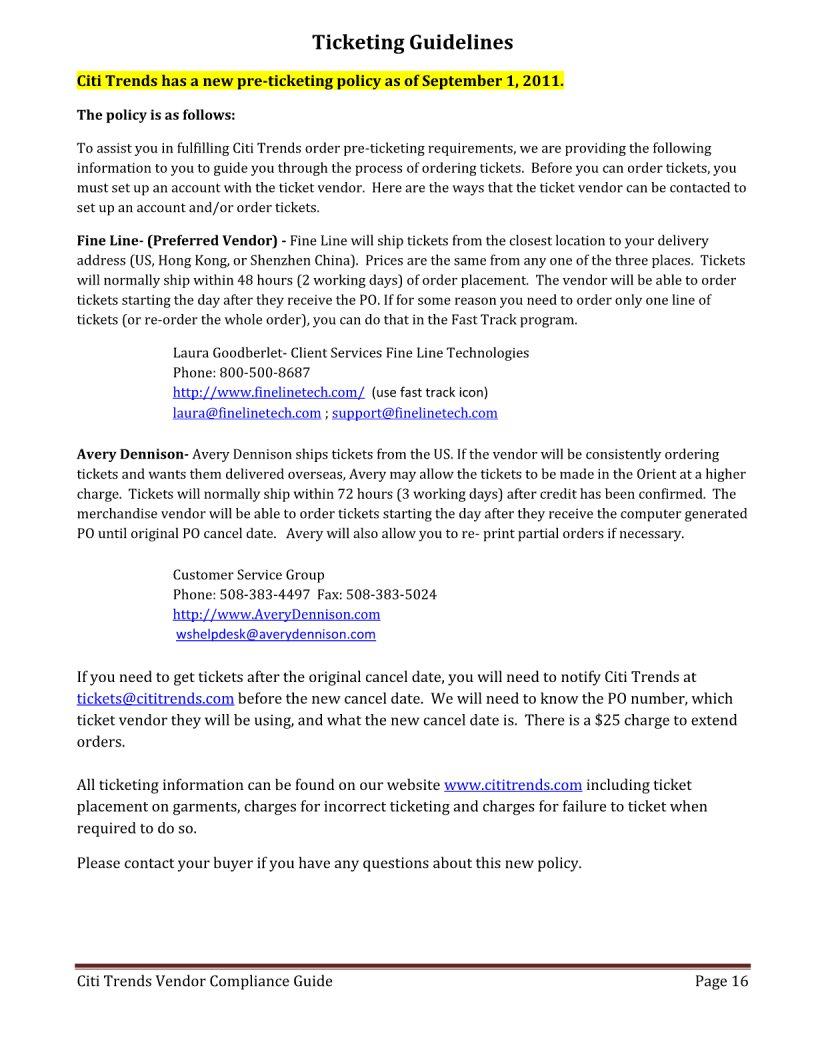This screenshot outlines the new pre-ticketing policy implemented by CityTrends effective September 1, 2011. To assist in meeting CityTrends' ticketing requirements, detailed guidelines are provided for ordering tickets. 

**Preferred Vendor: Fineline**
- **Account Setup**: Vendors must set up an account with Fineline to begin ordering tickets.
- **Locations**: Fineline ships tickets from the U.S., Hong Kong, or Shenzhen, China, with prices consistent across all locations.
- **Shipping Time**: Orders are typically shipped within 48 hours of order placement.
- **Order Process**: Fineline can process ticket orders starting the day after they receive the purchase order (PO).
- **Special Orders**: For single-line ticket orders, the FastTrack program is available.
- Contact Details: Includes the addresses, phone numbers, and email contacts for setting up accounts and ordering tickets.

**Alternative Vendor: Avery Dennison**
- **Account Setup**: Vendors can also set up an account with Avery Dennison.
- **Locations and Shipping**: Avery Dennison ships tickets primarily from the U.S., with a standard shipping time of three working days. They may also produce tickets in the Orient at a higher charge, contingent upon credit confirmation.
- Contact Details: Contains the customer service group's phone numbers and email addresses.

**Additional Notes**
- **Order Amendments**: If ticket orders need to be placed after the original cancellation date, vendors must notify CityTrends via a provided email.

This comprehensive guide aims to streamline the pre-ticketing process, ensuring compliance with CityTrends' policies.